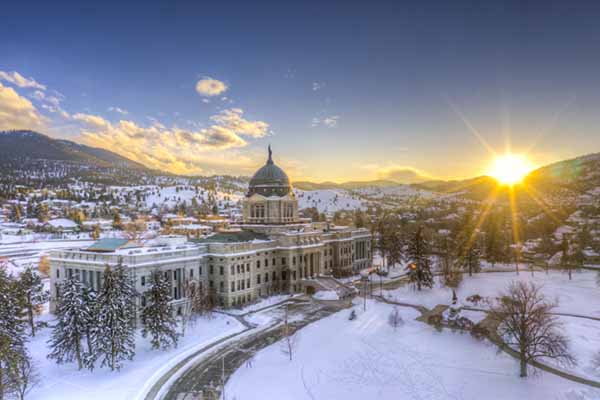This captivating photograph showcases a grand historical palace or parliament building enveloped in a winter wonderland. The majestic structure, likely about 200 years old and rising to four or five stories in height, features a striking blue-teal dome at its center atop a large, elegant staircase. The expansive estate stretches at least two to three hundred feet wide and is adorned with a circular drive-up driveway.

The building is set against a backdrop of towering, snow-covered mountains, emphasizing its prominence within the landscape. The scene is bathed in the warm, golden hues of a setting (or rising) sun, with a clear blue sky transitioning into the early or late day atmosphere. Puffy white clouds hover near the mountain peaks, gradually giving way to pristine, open skies.

The foreground of the image is blanketed in thick snow, dotted with bare trees and evergreen pine trees that frame the building. A well-defined footpath winds through the snowy gardens, enhancing the serene and picturesque quality of this winter scene. The overall ambiance is one of tranquility and historic grandeur, capturing the essence of a timeless winter moment in a mountain terrain city.